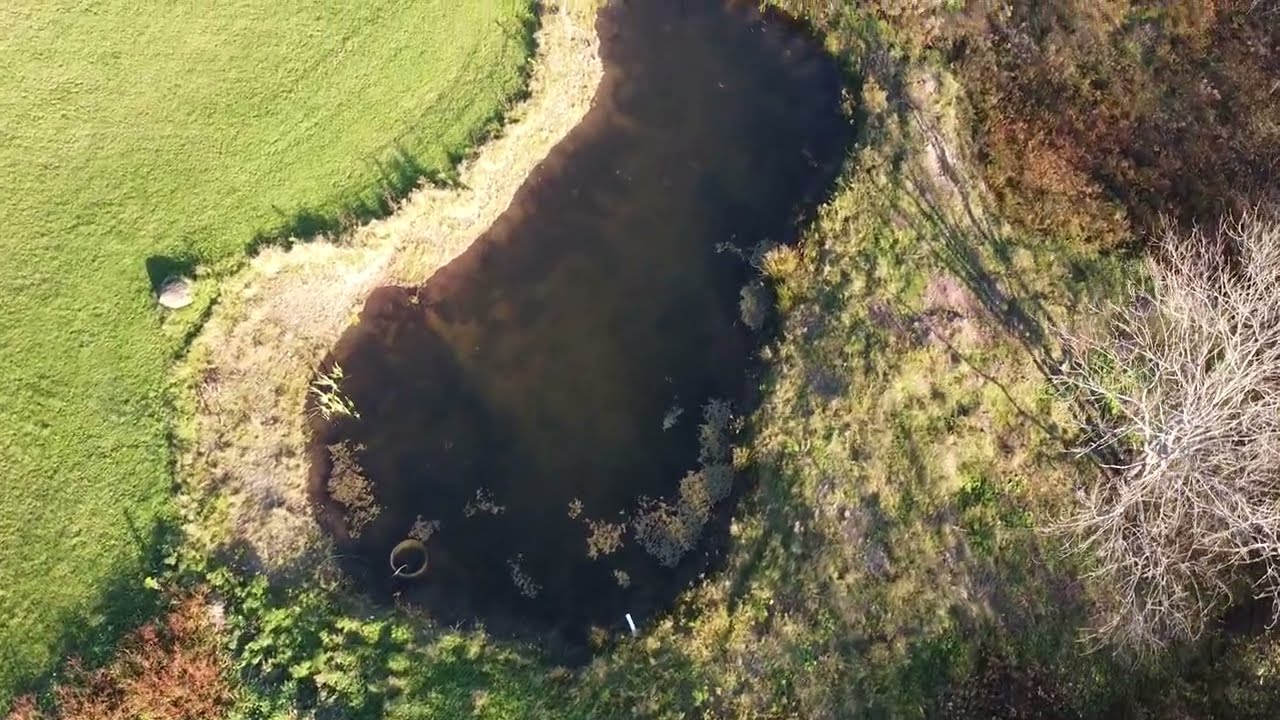This aerial, horizontally-aligned rectangular image showcases a diverse landscape centered around a bean-shaped pond with dark, murky brown water, interspersed with floating leaves. The pond extends from the top of the middle picture down to the bottom middle. 

To the left of the pond, there's a flat expanse of neatly trimmed, vibrant green grass, almost resembling a well-maintained yard or adjacent to a farm field. This grassy area gives way to a sandy shore as it approaches the pond. On the right side of the pond, the landscape transitions to a rougher terrain with some grayish, tan dirt and sparse shrubbery. Further right, there's a bare tree with gray branches, surrounded by fallen orangish leaves. In the upper right-hand corner, the ground appears rocky and brownish. Additionally, a round container can be spotted in the lower left part of the pond. 

The upper left side features more green grass, while the right side is marked by rocky ground and additional foliage. The image as a whole contrasts lush greenery with stark, barren elements, offering a detailed snapshot from an aerial perspective.